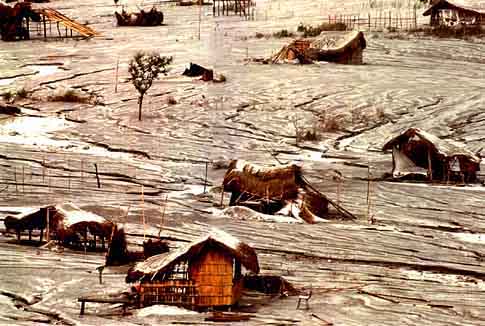This color photograph captures a desolate scene of a primitive village, seemingly devastated by a recent natural disaster. Central to the image are roughly half a dozen huts, largely constructed from bamboo and reeds, their roofs appearing to be made of grass or another natural material. Some huts feature porches and small added rooms, but they are largely caved in and damaged. The ground is a mix of brown mud, water, and patches of snow, giving the setting a bleak and chaotic appearance. A prominent house in the foreground has reddish wood siding, a grass-thatched peaked roof, and a porch on the left. Surrounding the homes are thin sticks, possibly used to demarcate pathways or mark a road. A single tree stands amidst the ruined village, adding to the eerie quietness of the scene. The entire landscape appears as though it has been ravaged by a flood or some storm, with flowing mud and water stretching into the distance, and the sepia tint suggests an aged, historical quality to the image.